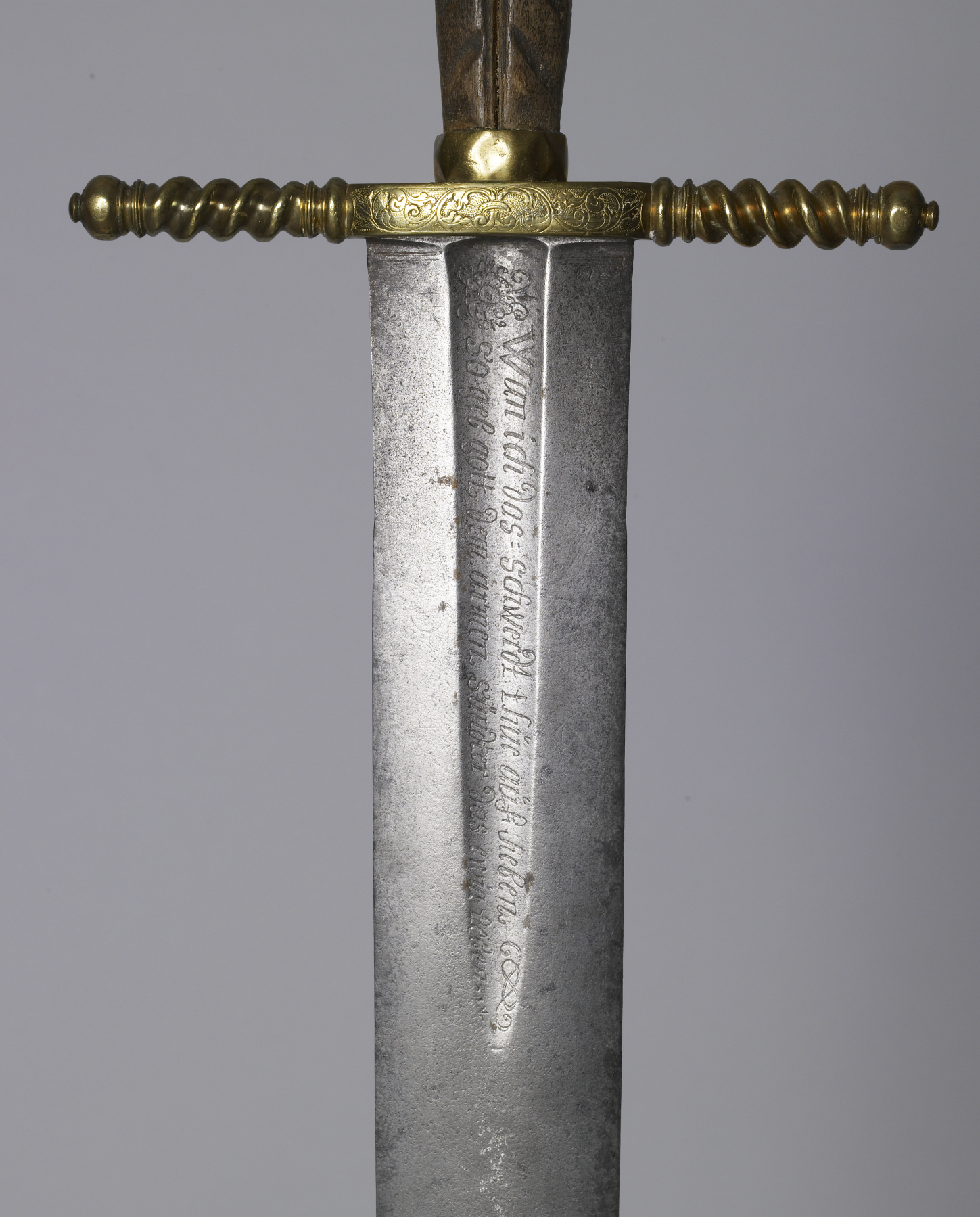This image is a detailed, color photograph in portrait orientation, showcasing a close-up view of a sword. The background is a solid gray with subtle shading, likely from illumination. The sword is positioned vertically, extending beyond the top and bottom edges of the image, with only a portion of the handle and blade visible. The handle, part of which is cropped out, is black and features a small screw or nail where it attaches to the blade. The crossguard is a brass or gold-colored horizontal piece with rounded knobs at the ends and a spiral coil pattern wrapped around it. The blade, made of silver metal, appears worn and used with an indentation that runs from the base down about three-quarters of its length. There are faint, unreadable engravings in a foreign language along this indentation. The overall style of the image leans towards photographic realism, capturing the intricate details and textures of the sword.